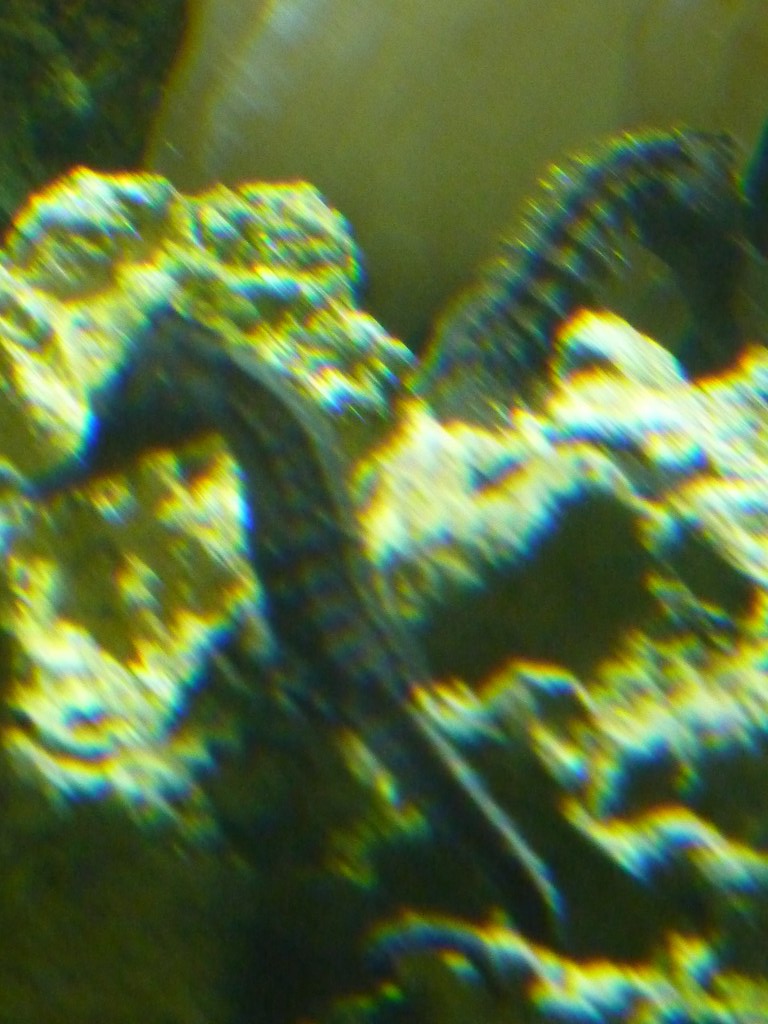This color portrait-mode photograph, despite its poor quality and out-of-focus nature, captures two seahorses against a textured, beige rock formation. The image is close up, with one seahorse prominently positioned in the foreground. This seahorse stands mostly upright, its head angled downwards and to the left, displaying its long, flat snout and textured skin. In the background, another seahorse faces downward and to the right, partially obscured by the greenish-yellow, rough-looking rocks. The lighting in the photo is dim, adding a dark blue and yellow striped effect to the rocks and creating an overall more muted color palette. The upper left-hand corner of the image is darker, though any specific details are indistinguishable.